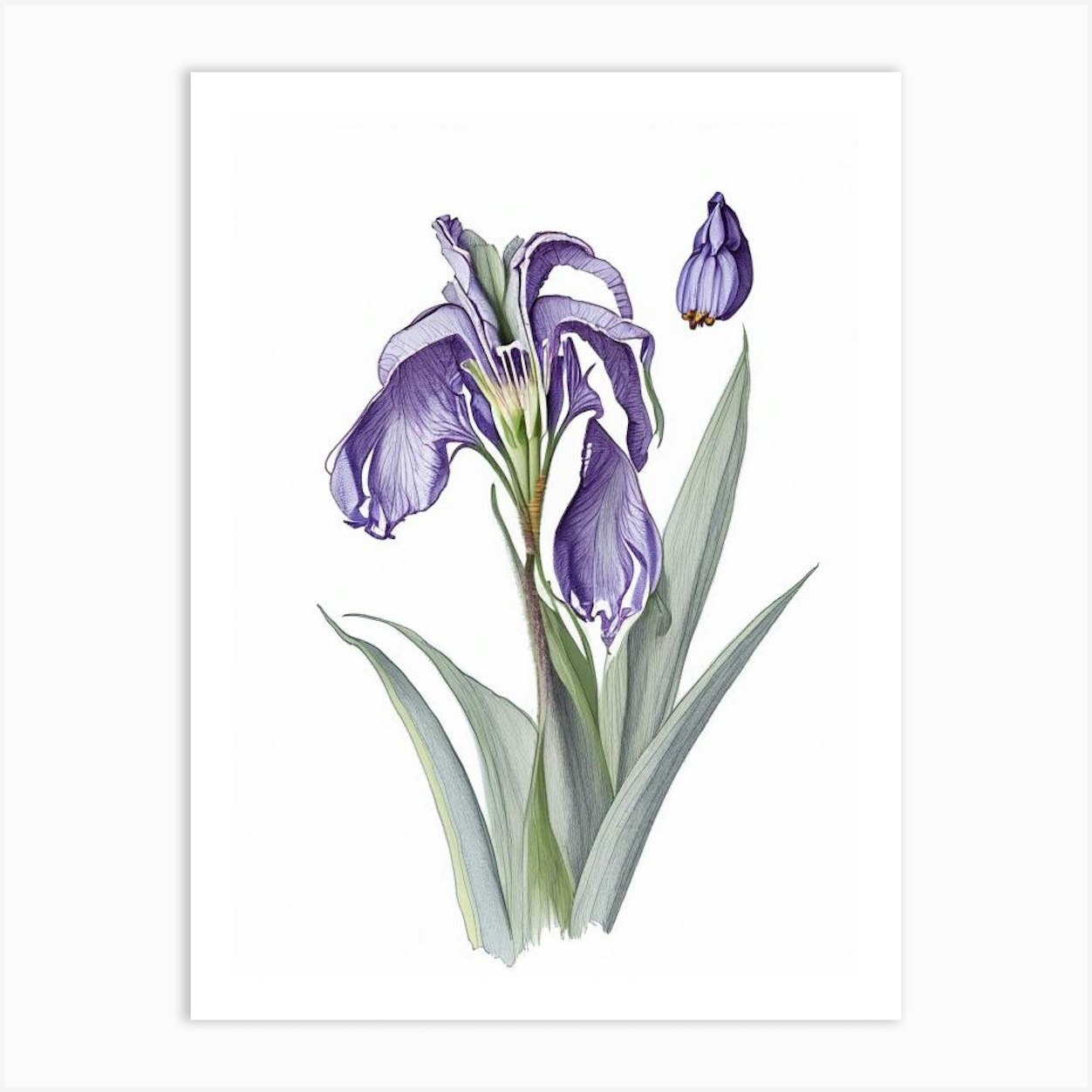The image features a hand-sketched graphic of a plant, most likely an iris, prominently displayed against a stark white background. The plant is centered and upright, with six large, spiky leaves that transition from dark green at the bottom to lighter green towards the top. A tall stem rises from the middle, supporting a striking light purple flower composed of six petals with white accents. To the right of this main flower, there appears to be a partially shown, separate flower, possibly an undeveloped bud. The flowers exhibit detailing that includes tiny yellow bits at the tips. The background of the image consists of an off-white rectangle, within which is a smaller white rectangle resembling a piece of paper or canvas, giving the composition a classical and flat appearance, akin to a delicate pen or pencil sketch rather than a watercolor.